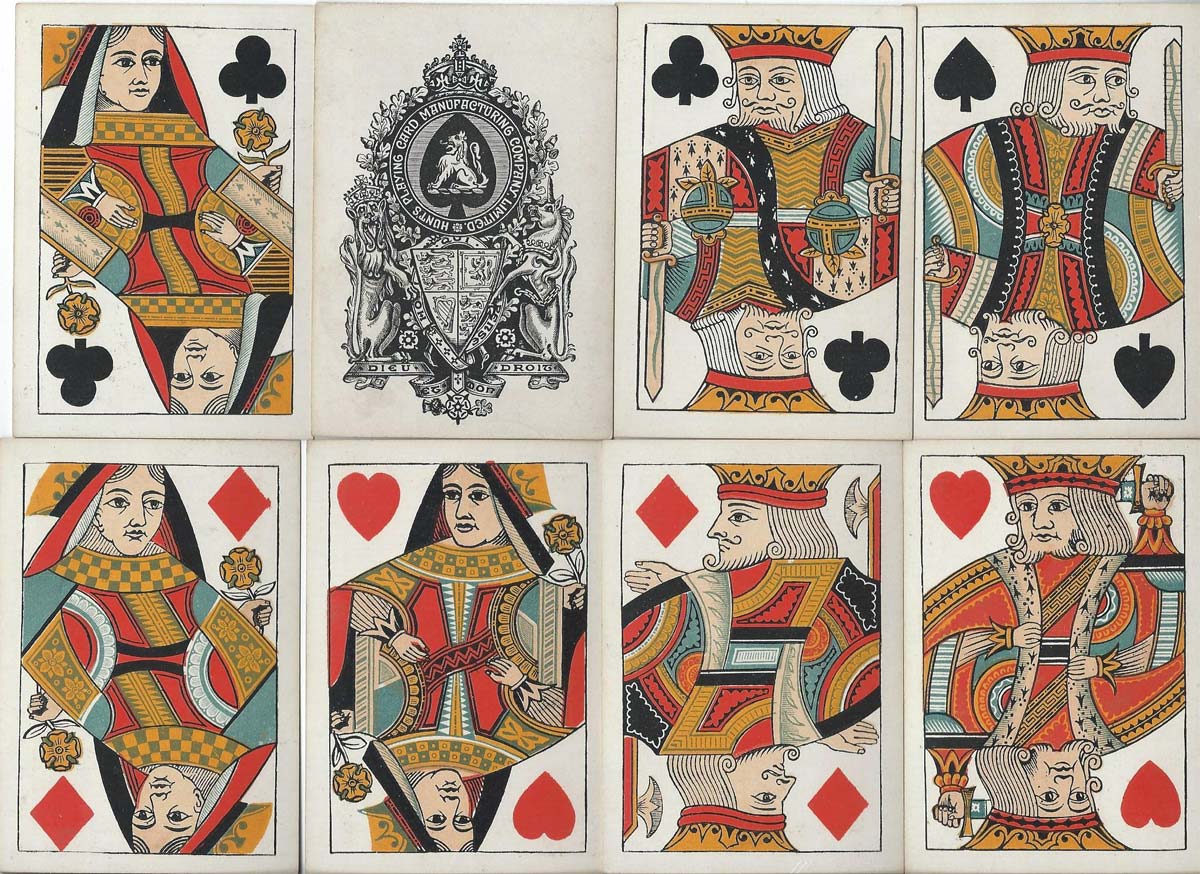This photograph showcases a set of eight playing cards arranged in two rows of four on a white background. Each card features a distinct face or intricate design. Starting from the top left, the first card is a Queen of Clubs, beautifully illustrated within a white border outlined by a thin black line. Next to it is the back of a card, adorned with an elaborate crest featuring a crown, two horses, and a central lion enclosed in a circle, accompanied by the inscription "Playing Card Manufacturing Company Limited Hunts" in white text. To its right, the third card is a King of Clubs, followed by a King of Spades. In the second row, from left to right, there's a Queen of Diamonds, a Queen of Hearts, a King of Diamonds, and finally, a King of Hearts. The face cards are elegantly rendered in vibrant blacks, reds, and hints of gray, capturing the essence of classic card royalty.